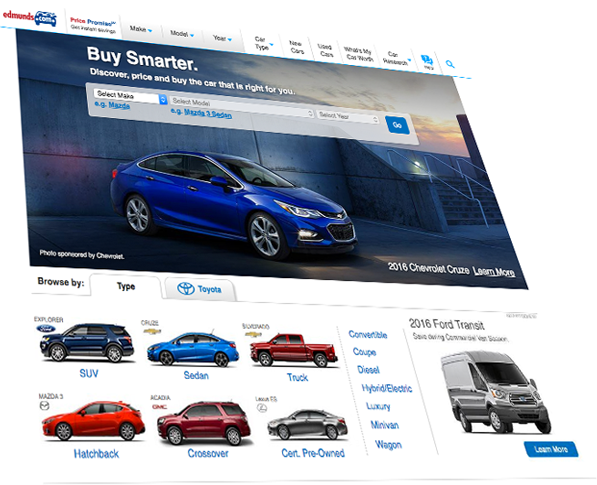The image is a slanted screenshot from the website Edmunds.com, tilted slightly backwards to the left. At the top, a white banner displays "Edmunds.com" with the car headlights creatively forming the 'O' in ".com". Next to it, the text "Price Promise" is visible. The website features different options, including a download button and a dropdown menu, though the diagonal slant makes them difficult to read.

In the middle section, there's an outdoor image featuring the right side of a blue car. The text "Buy Smarter" appears in bold white print above the message, "Discover, Price, and Buy the car that is right for you."

Below this, a banner presents a dropdown menu with options labeled "Select Make (e.g., Mazda)," "Select Model (e.g., Mazda 3)," and a call-to-action button that reads "Go."

Lower down, a white background segment categorizes browsing options by vehicle type. The section starts with "Browse By Type" and includes types like Hatchback, SUV, Sedan, Crossover, Truck, and Certified Pre-Owned. Among the vehicle manufacturers listed are Toyota, Lexus, Chevy, GMC, Mazda, and Ford. 

On the left sidebar, additional categories include Convertible, Coupe, Diesel, Hybrid/Electric, Luxury, Minivan, and Wagon. 

Towards the bottom, there's an image and description of a 2016 Ford Transit van.